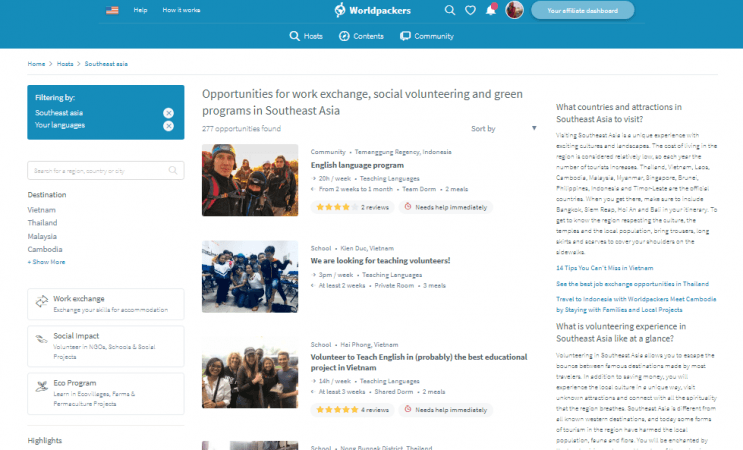Here's a detailed and cleaned-up caption for the described image:

---

The webpage features a dark blue bezel at the top. On the left-hand side, an American flag is presented with adjacent white text that reads "Help." Next to this, there are two buttons labeled "Help" and "How It Works." Centered prominently in bold white text, a globe tilted to the right with an axis through it is labeled "World Packers." To the right of the logo, there is a search icon, a heart icon, and a notification bell with a red indicator signifying new notifications. 

A profile picture of a user is displayed next to a raised cyan blue button with white text that reads "Your Affiliate Dashboard." Below this section, a variety of programs and opportunities are showcased. At the top, a list highlights work exchange, social volunteering, and green programs in Southeast Asia, alongside an image of a group of people hiking outdoors captioned "English Language Program." Another image depicts individuals inside a gymnasium with a label "We Are Looking for Volunteers." Further below, a crowd near a tree line is captioned "Volunteer to Teach English" with an added note proclaiming it as "probably the best educational project in Vietnam."

On the right-hand side, a text block provides travel and volunteer information, though some parts are blurred. Visible text includes hyperlinked titles like "16 Tips You Can't Miss in Vietnam," "See the Best Job Exchange Opportunities in Thailand," "Travel to Indonesia with World Packers," and "Meet Cambodia by Staying with Families and Local Projects."

To the left, several clickable buttons are seen— "Home," "Host," and "Southeast Asia." Below these, a dark blue rectangle with "Filtered By" in white text lists "Southeast Asia” with an “X” in a white circle to its right, indicating filter options followed by another for languages. 

Further down, there's another gray-text search bar, unreadable in detail, accompanied by a magnifying glass icon. Underneath, text "Destination" is followed by blue hyperlinked text for Vietnam, Thailand, Malaysia, and Cambodia, with a “+ Show More” option for additional destinations.

Additionally, three black text rectangles list program categories: "Work Exchange," "Social Impact," and "Eco Program." At the bottom left, a segment titled "Highlights" begins to introduce another program, though it is partially cut off.

---